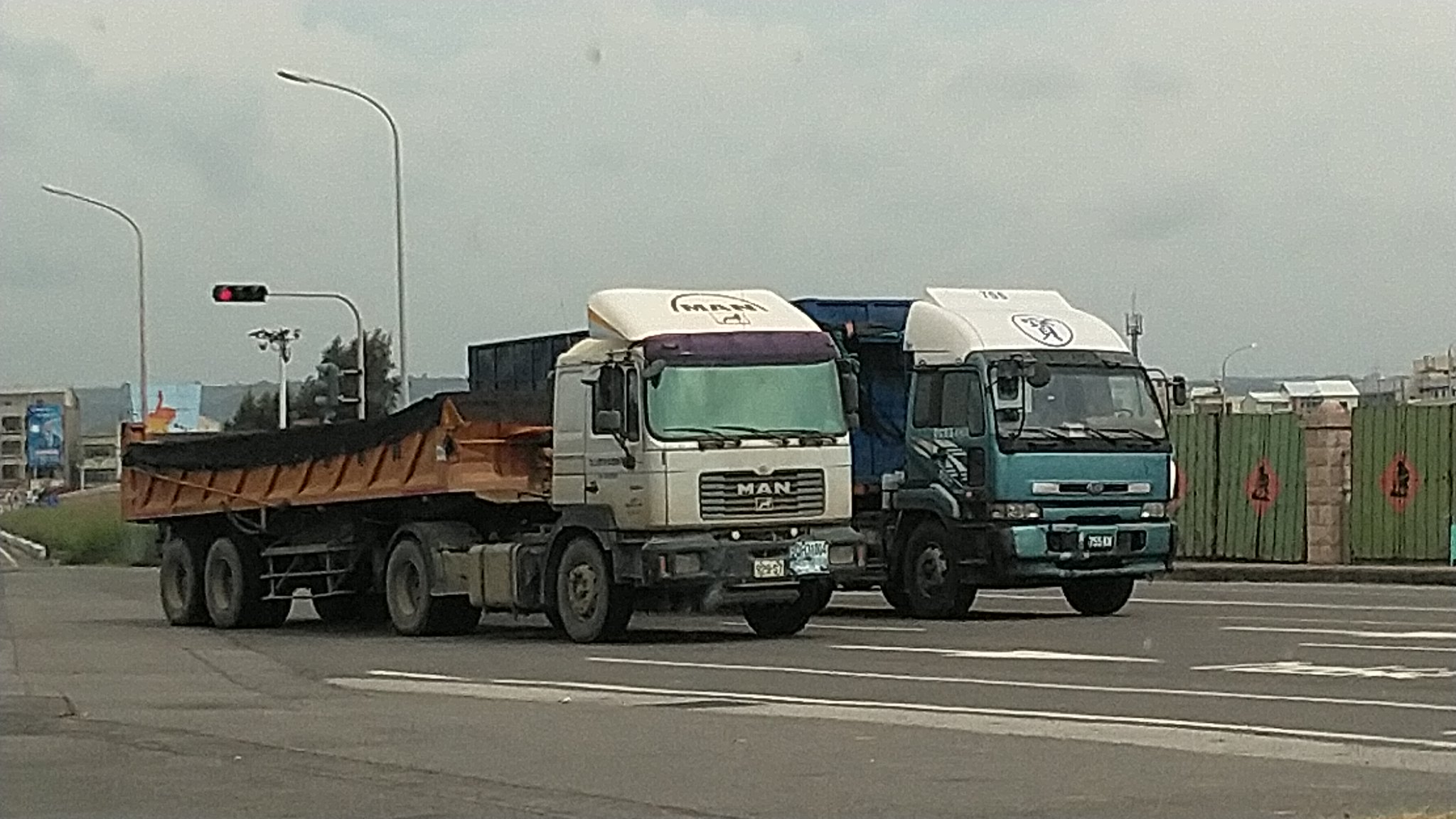This outdoor color photograph captures two large semi-trucks side-by-side on a multi-lane highway during an overcast, hazy day. Dominating the center of the image, these cab-over trucks appear to be stationary, absent of visible drivers. The truck on the left features a white cab with the logo "MAN" prominently displayed on its grill. This truck pulls a dump trailer with two axles, its cargo obscured by a large black tarp, and the trailer is dark orange in color. Meanwhile, the truck on the right has a teal-colored cab with a heart and number "756" as part of its logo, and it pulls a blue box trailer container of standard height, suggesting a secure load.

Both trucks occupy nearly the entire frame and are positioned parallel to each other. Above the scene, a traffic light displays a red signal near the top left, accompanied by two street lamps. In the background, beyond a fence on the right, the hazy outline of a cityscape emerges, adding depth to the scene. This meticulous alignment of vehicles and urban elements draws focus to the trucks' imposing and somewhat enigmatic presence on the road.